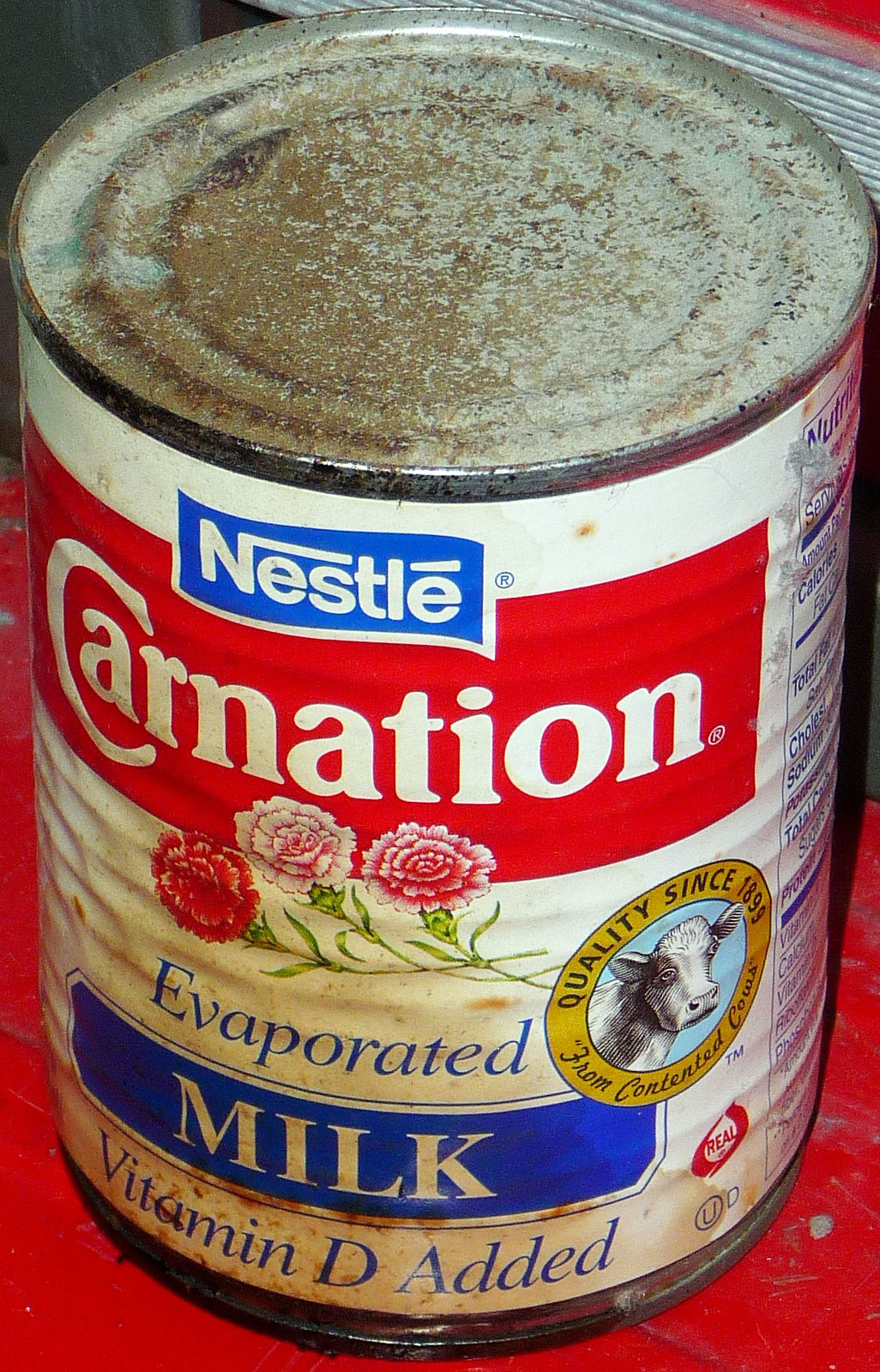The image displays a close-up of a very old, rusted can of Carnation evaporated milk with vitamin D added. The main label is mainly white with accents of red and blue, and it features the iconic Nestlé logo in white and blue. The front of the can prominently displays the word "Carnation" in white against a red background, accompanied by an illustration of three carnations at the bottom center. Just below the flowers, the label states "Evaporated Milk, Vitamin D Added" in blue and white text. On one side, there is a nutrition label, and the other side features a circular drawing of a cow's head with the phrase "Quality Since 1899" from contented cows. The label is discolored, reflecting the can's significant age, suggesting it has been long forgotten on a shelf or in storage.